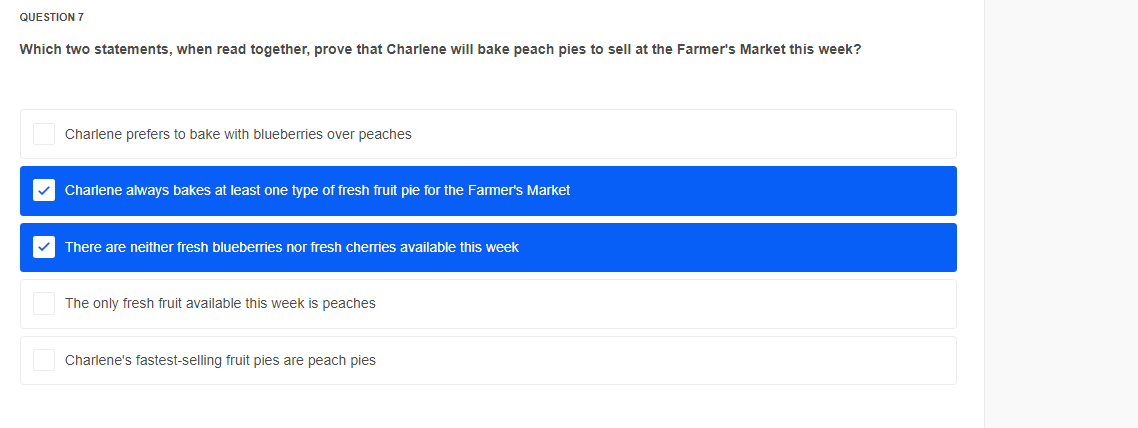The image depicts a section of a website, specifically starting at question seven, indicating that it is mid-way through a series of questions. The heading in the upper left-hand corner reads "Question 7." The question presented is: "Which two statements, when read together, prove that Charlene will bake peach pies to sell at the farmer's market this week?"

The question includes five multiple-choice statements:

1. "Charlene prefers to bake with blueberries over peaches."
2. "Charlene always bakes at least one type of fresh fruit pie for the farmer's market." This statement is in a blue box with a small white checkmark.
3. "There are neither fresh blueberries nor fresh cherries available this week." This statement is also in a blue box with a small white checkmark.
4. "The only fresh fruit available this week is peaches."
5. "Charlene's fastest-selling fruit pies are peach ones."

The selected answers are statements two and three, as indicated by the checkmarks in the white boxes beside them. These boxes are highlighted in blue, clearly showing they have been chosen as the answers.